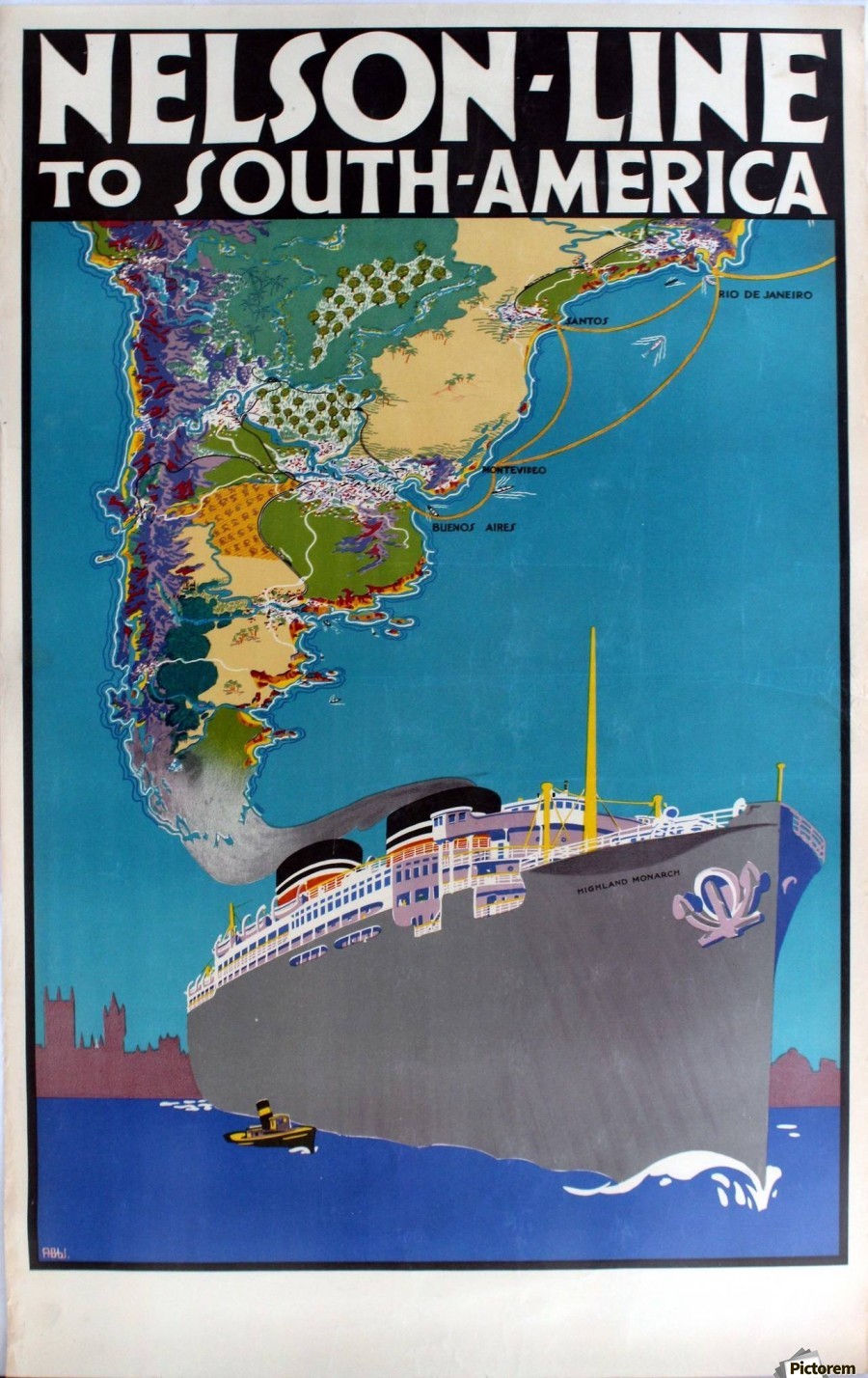The image is an elaborate and colorful vintage advertisement for the Nelson Line cruise route to South America. Dominating the upper section of the poster is a heading in white text on a black background that reads "Nelson Line to South America." Directly below, a detailed and vibrant map of the southern part of South America displays countries such as Brazil, Chile, and Argentina, highlighted in an array of yellows, greens, purples, and blues, against a blue background symbolizing the ocean. 

The poster artistically blends into the scene where an imposing gray steamship with white and blue details sails below the map. The steamship features multiple levels, blue windows, white outer decking, and is equipped with two large smoke stacks, billowing smoke that blends into the cloudy sky, through which the map of South America appears to merge seamlessly.

The bottom of the ship, painted gray, cuts through the blue water, creating white waves. Adjacent to this steamship is a smaller yellow and black boat. The lower background showcases a skyline of prominent pink buildings, reminiscent of a cityscape perhaps suggesting destinations like Buenos Aires, Montevideo, Rio de Janeiro, and Santos, as notated on the map.

Overall, the poster exudes an old-world charm, merging geographical details with the romance of sea travel, aiming to captivate potential passengers with its rich colors and promise of South American adventure.